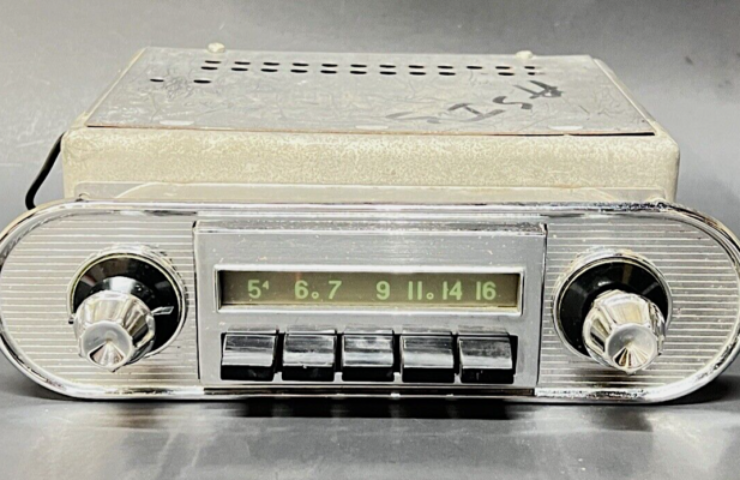This image shows a vintage car radio, likely from the 1940s. The radio has a distinctive oval form with rounded edges and is primarily silver in color. On the front, there are two metal knobs, one on each side, encircled by black plastic rings. Between these knobs, there is a display area featuring radio frequencies, with lime green digits set against a black background. Below the display, five chrome-colored buttons are aligned, which likely allow for preset station selection. The frequency dial includes numbers that begin at 5 with an arrow, followed by 6, 7, 9, 11, 14, and 16, separated by varying spaces. The back of the radio shows a box-like structure containing its electronics, with punched holes serving as vents and some alphanumeric writing, possibly “A-S-I-J.” There is also a wire protruding from the rear of the unit. The radio is placed on a gray surface against a similar gray background, highlighting its vintage design and detailing.